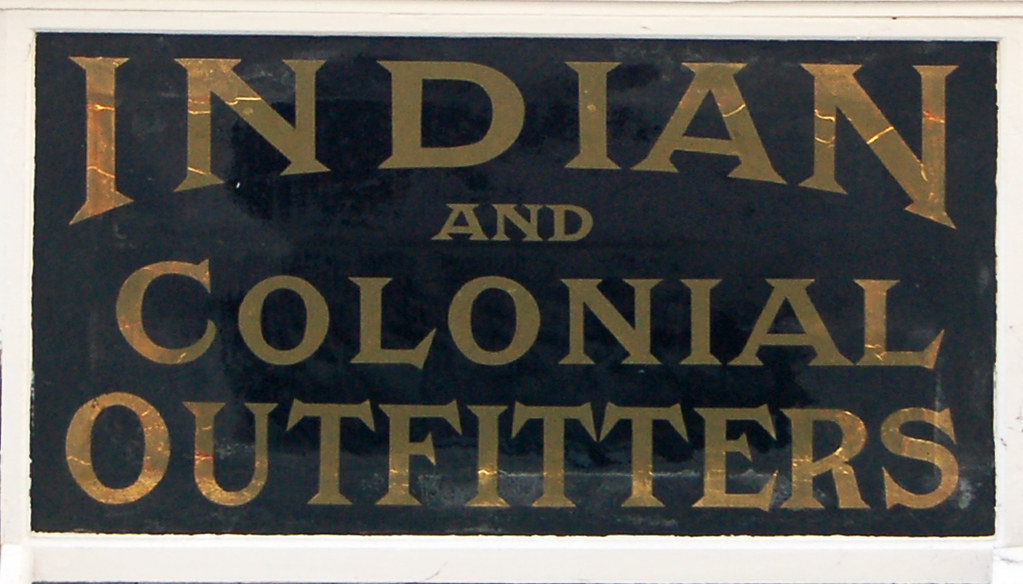The image features a photograph of a rectangular sign, which appears to be taken through a window or with a piece of glass in front, giving it a slight reflective quality. The sign is framed in mitered white wood, with a black background. The text on the sign is in shimmering gold font, with "Indian" at the top, followed by a smaller "And," and then slightly larger "Colonial Outfitters" below it. There is also a faint silhouette image either reflecting on the glass or the black background, adding to the overall reflective appearance.